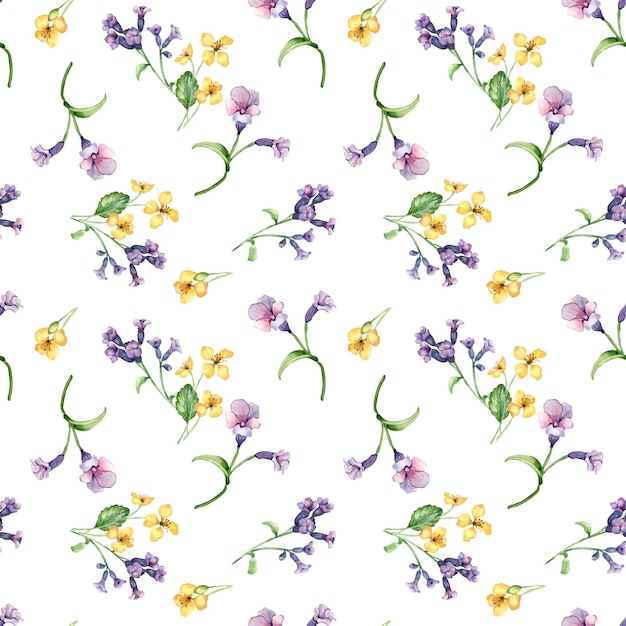The image depicts a vintage-patterned wallpaper or poster with a seamless, repeating tile pattern of dainty flowers on a solid white background. The design features small purple and yellow flowers with green leaves and stems. The purple flowers often appear in pairs, with one flower fully open and another barely open, while the yellow flowers vary between single blossoms and clusters of three. Each flower is intricately detailed, with some having round centers and others featuring wispy offshoots. The harmonious arrangement of the flowers, green stems, and leaves creates an elegant and symmetrical pattern, reminiscent of a traditional, perhaps nostalgic, design.